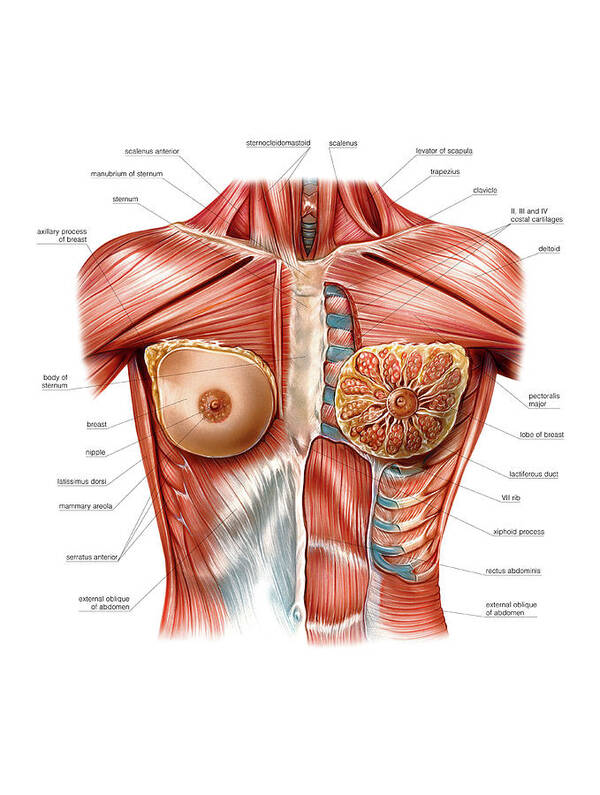This is an illustration of the upper portion of the human anatomy, focused primarily on the muscular system. The diagram is cut off at the neck, displaying a small part of the neck and the shoulders, and extends just below the waist, capturing the entirety of the torso. The inner structures of the body are exposed, with no skin visible, emphasizing the various muscle groups. The ribcage is prominent, contributing to the grounded understanding of the anatomical layers. The entirety of the torso is depicted in shades of red, highlighting the muscles. Labels with corresponding lines are carefully positioned, pinpointing and identifying the different muscles and anatomical features in the image.